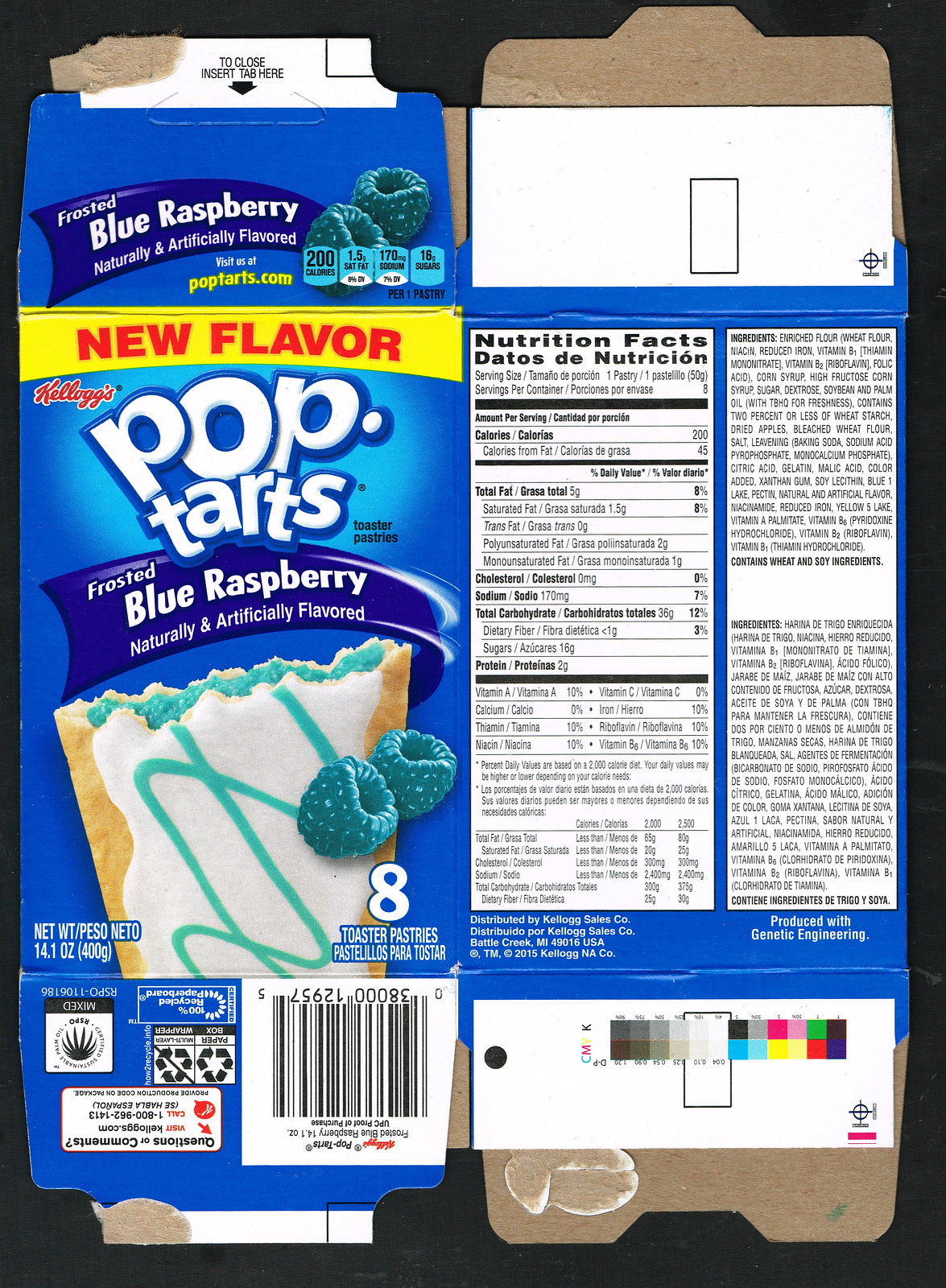This image showcases a package of Kellogg's Pop-Tarts, specifically highlighting the "Frosted Blue Raspberry" flavor, which is a new addition to the product line. The package has been flattened, allowing a full view of both the front cover and the nutrition facts on the reverse side. The front cover prominently displays the Kellogg's branding along with text that reads "Frosted Blue Raspberry Naturally and Artificially Flavored." 

A vivid illustration of the Pop-Tart can be seen, depicting its blue raspberry filling encased in a pastry topped with white icing and a blue swirl design. The imagery also includes blue raspberries, emphasizing the flavor. The package notes that it contains eight toaster pastries, with a total weight of 14.1 ounces. 

Additionally, the detailed nutrition facts are presented, including information on the saturated fats, calories, ingredients, and other nutritional components, which are also listed in Spanish. This comprehensive view provides all the necessary details about the contents and nutritional value of the Pop-Tarts.